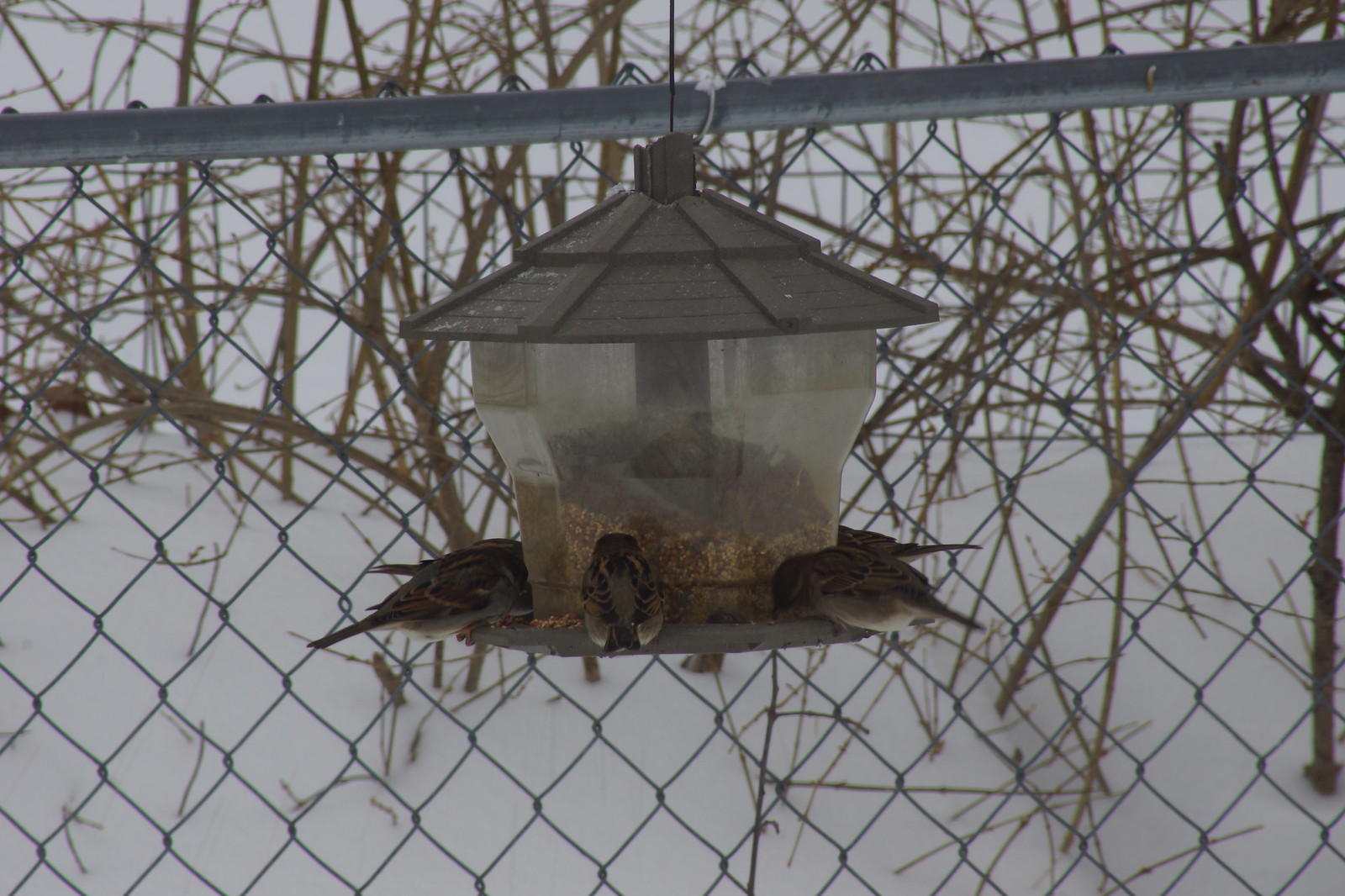In the photograph, a winter scene unfolds with a bird feeder taking center stage. Hanging from a seemingly invisible support, the feeder is shaped like a small hut with a transparent portion revealing it to be about a third of the way full with seeds. Five small, dark brown birds with white bellies are energetically feeding from it, their presence adding life to the dreary day. The background is dominated by a chain-link fence intertwined with bare brown branches, possibly brambles, and further back, another layer of a fence, potentially made of chicken wire, is just visible. The ground is blanketed with snow, the overall atmosphere gray and overcast, yet the lively activity at the feeder provides a quaint and heartwarming focal point amid the wintry landscape.